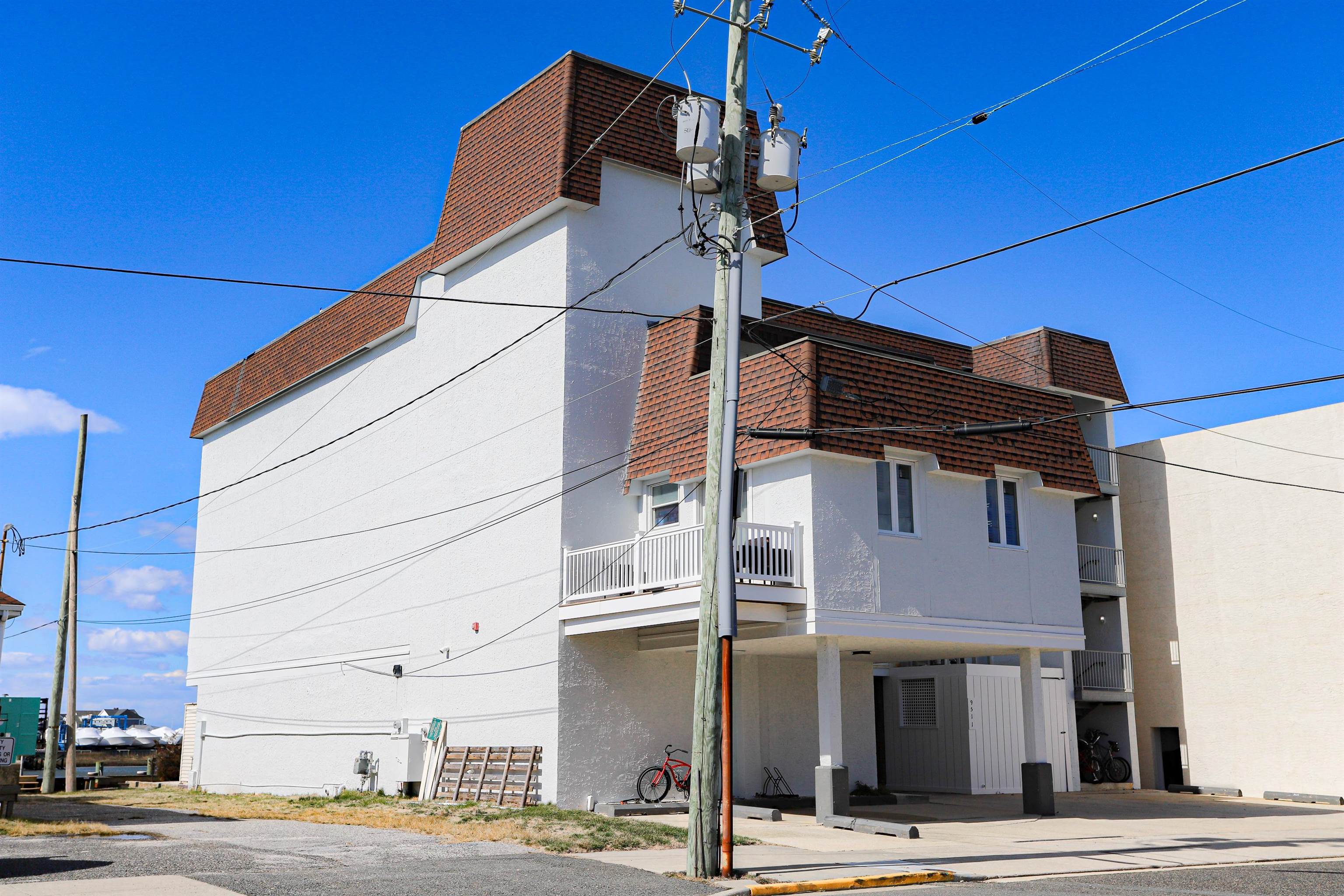The photograph captures a clean, multi-level white building with a reddish-brown roof, situated amidst other structures in a cityscape. Prominently featured are the front and side views of the building, which includes a second-level outdoor patio and a front-facing staircase. The building appears residential, perhaps an apartment. Two windows are visible on its façade. 

In the foreground, a red bike rests against the building, and nearby are some wooden pallets and assorted debris along the side. Centered within the image is a utility pole festooned with wires stretching across the scene, suggesting strong electrical service connectivity. Another orange pole stands adjacent to it. A blue sky with sparse clouds dominates the background, indicating a sunny day. There is also an intriguing hint of what might be boats visible in the left-hand corner.